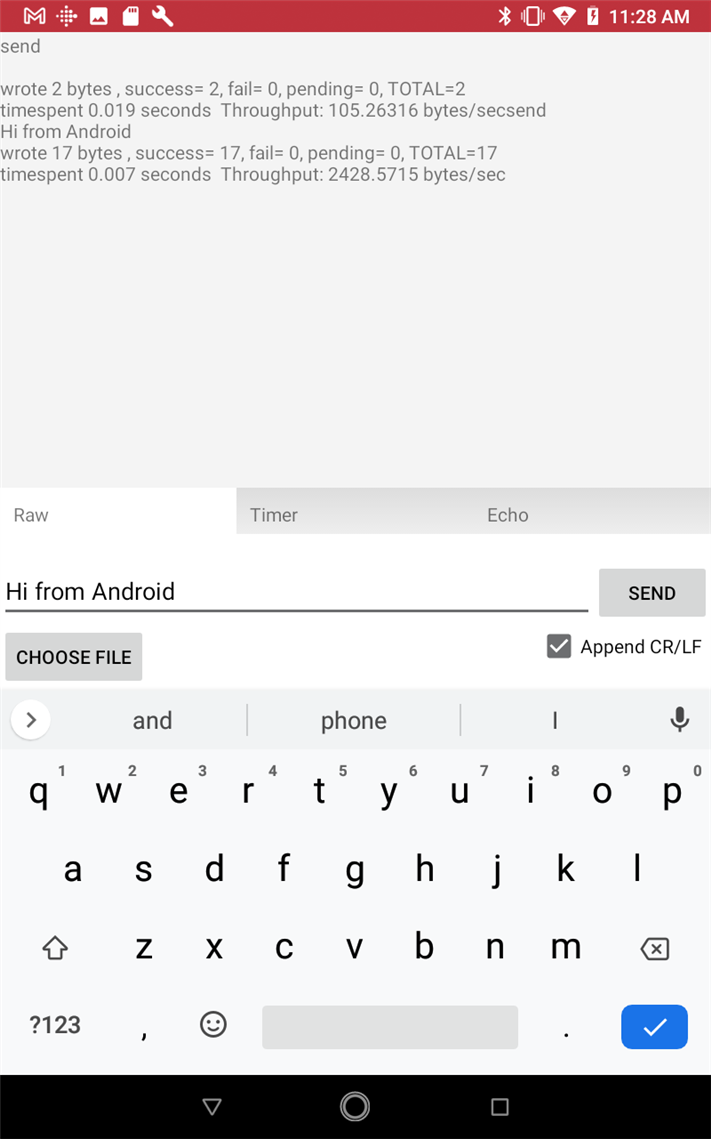This is a detailed caption of the image that was described:

---

The screenshot is of a message interface on a mobile device. At the top of the screen, there is a red stripe that contains several icons. On the left side, there are a mail icon and a wrench icon. On the right side, the screen displays the time "11:28 a.m.," along with icons for battery life, Bluetooth connectivity, and a vibrating mobile indicator.

The main body of the webpage is gray, featuring darker gray text sections. The text includes the following details: "send row 2 bytes, success = 2, fail = 0, pending = 0, total = 2, time spent = 0.019 seconds, throughput = 105.26316 bytes/second." Continuing on, another section reads: "sent 'hi from Android', wrote 17 bytes, success = 17, fail = 0, pending = 0, total = 17, time spent = 0.007 seconds, throughput = 2428.5715 bytes/second."

At the bottom of the screen, there are three tabs labeled "Raw," "Timer," and "Echo," with the "Raw" tab currently selected. Under the "Raw" tab, there is a line of text that reads "hi from Android." Beneath this, there are buttons labeled "Choose File" and "Send File" on the right side, with a checkbox labeled "Append CR/LF" next to them. Finally, at the very bottom of the screen, a QWERTY keyboard is visible.